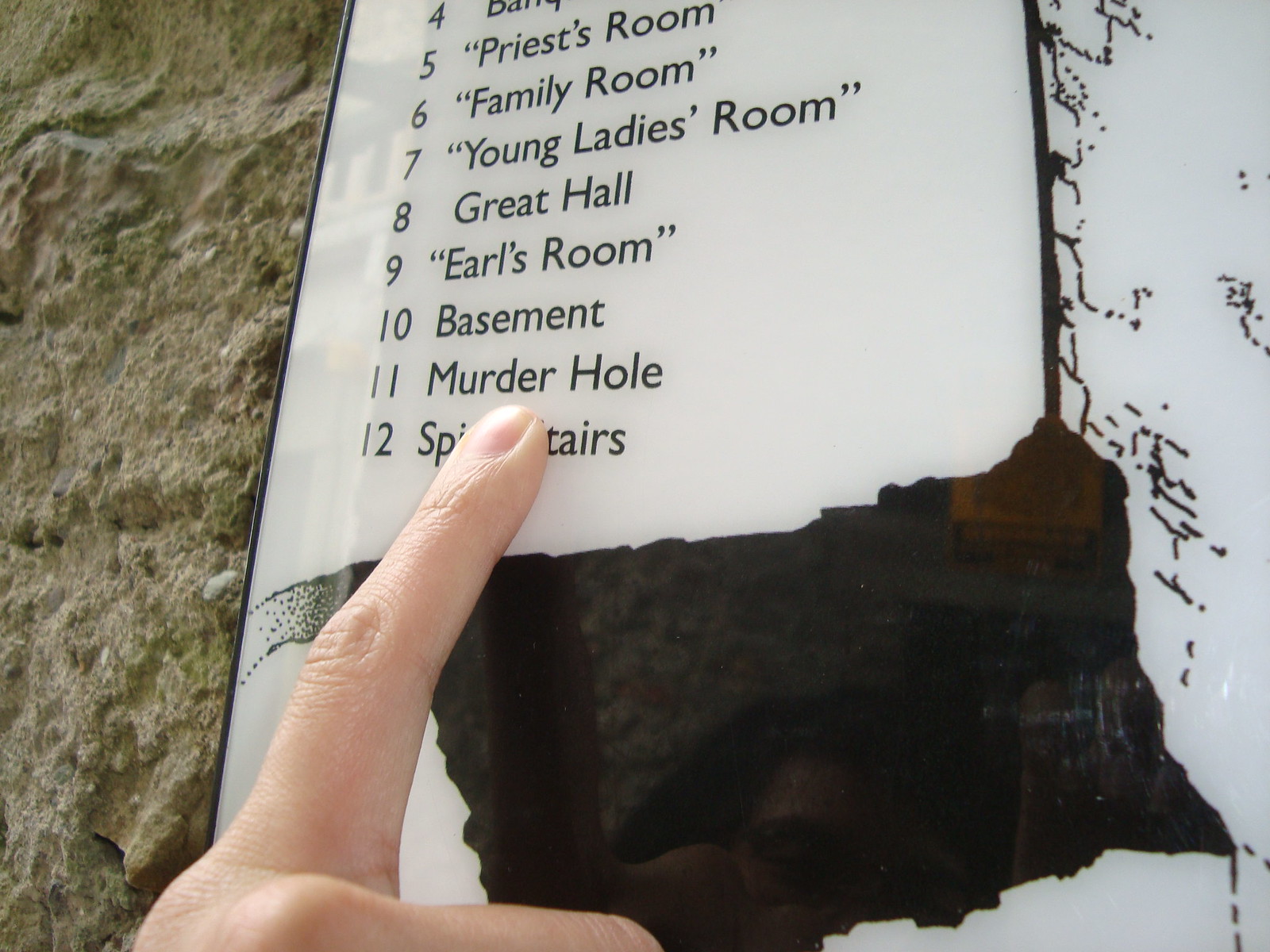This photo shows a glass-framed informational placard mounted on a rocky wall, likely representing a map of a building. The placard features a black illustration of a tunnel or cavern with a reflective surface. The list on the placard enumerates locations within the building, partially obscured but including, "4. Banquet Hall," "5. Priest's Room," "6. Family Room," "7. Young Lady's Room," "8. Great Hall," "9. Earl's Room," "10. Basement," "11. Murder Hole," and "12. Spiral Stairs." A person's finger, reflected in the black illustration, points almost touching number 11, labeled "Murder Hole."